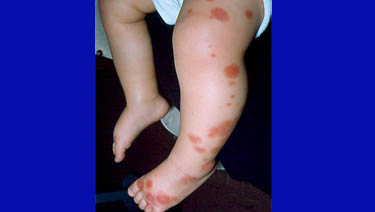The image is a vertically cropped photograph focused on the legs of a young child, possibly a baby around one to two years old, with light pale skin. The child appears to be wearing a diaper, and the background is a solid black color, framed by two large dark blue stripes on either side, indicating the image has been edited to spotlight the legs. The left leg is notably marked with blotchy, red-pink patches, indicative of a severe skin condition, allergic reaction, or rash, while the right leg appears clear. The contrast between the white skin and the inflamed patches on the left leg is stark, making the condition easily visible. The image is bright and clear, likely used for medical purposes such as diagnosis or educational training for young practitioners. There are no additional elements like text or other individuals in the photograph, ensuring the focus remains solely on the child’s affected legs.